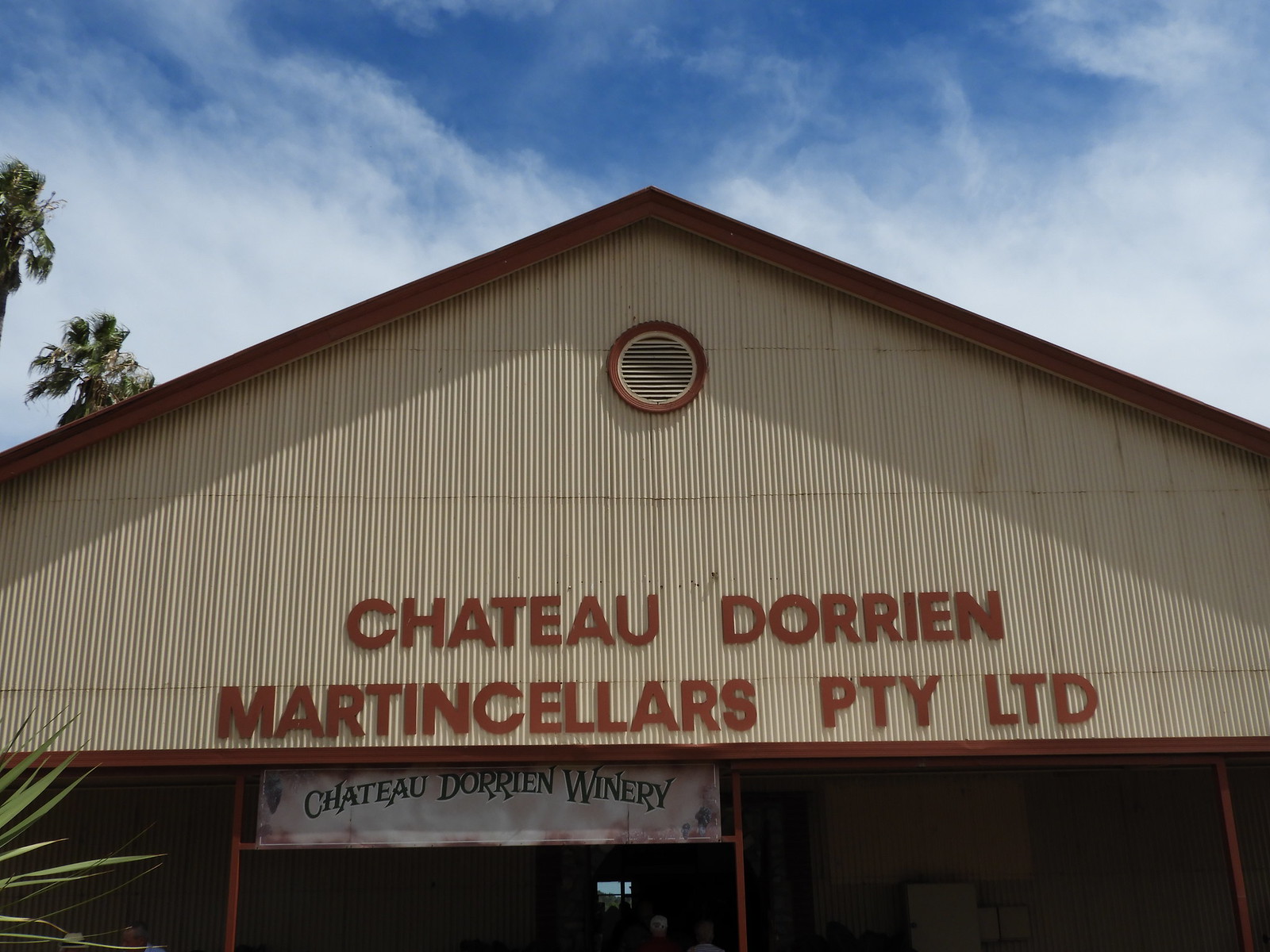The photo showcases the upper portion of a building taken during the daytime, featuring a brown and white facade. Prominently displayed on the side of the rooftop are signs that read "Chateau Dorian Martin Sellers Pty Ltd," indicative of a winery, as further confirmed by a white banner with black writing underneath the roofline that reads "Chateau Dorian Winery," supported by brown poles. The rooftop is adorned with brown and beige wood-like vertical structures. The outdoor setting reveals a blue sky with wispy white clouds and tall palm trees which extend above the roofline, positioned both in the foreground and background to the left. Additionally, an open doorway is visible at the front, with people standing inside, hinting at more activities within the building. Peeking through the doorway, one can spot a window on the opposite side and what appears to be a refrigerator positioned outside in front.